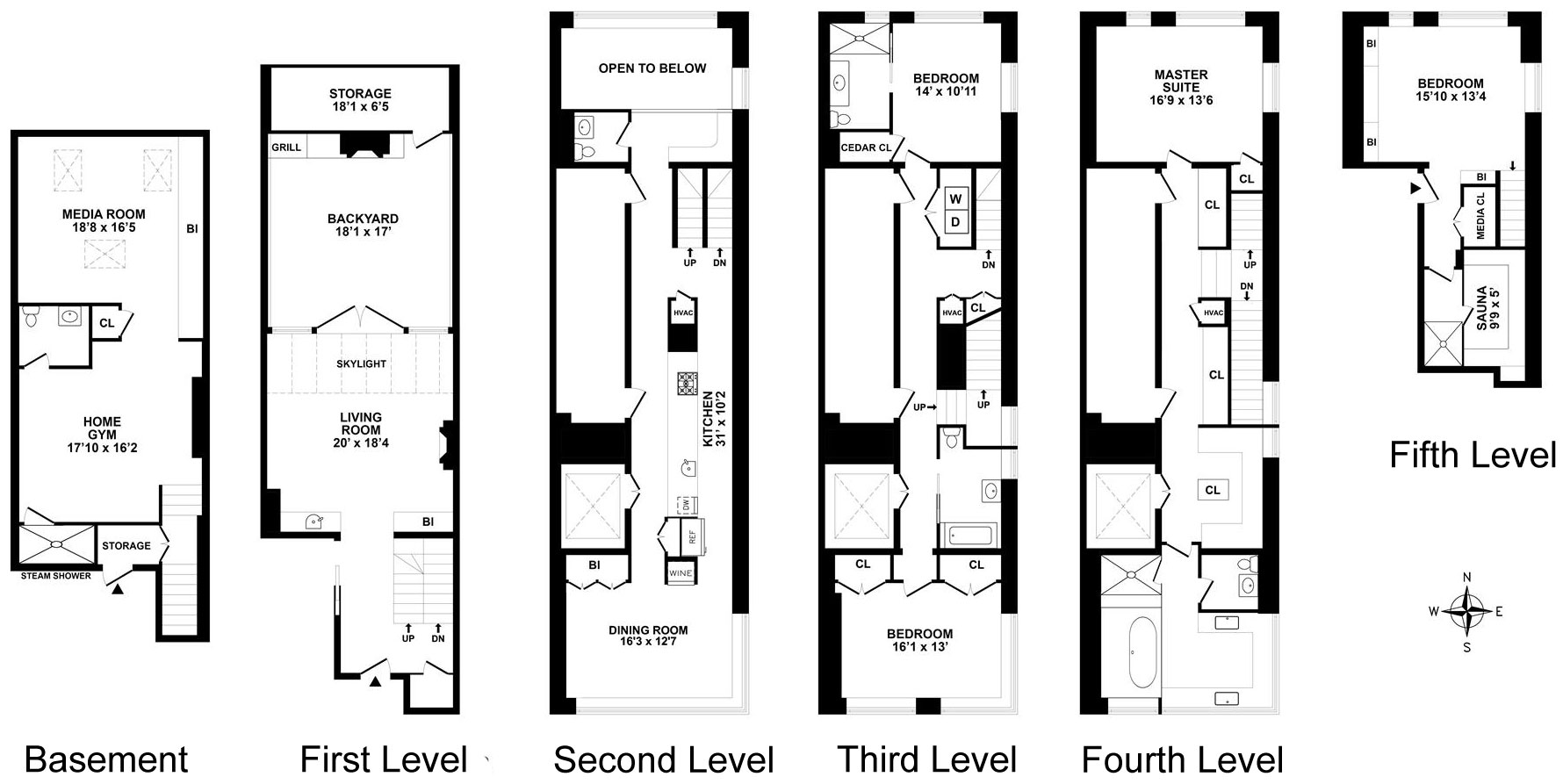The image showcases detailed blueprints of a multi-level house designed by a draftsman. The plans are in black and white and outline the layout across six distinct levels:

1. **Basement Level**: Features a media room at the top with specified dimensions, and a home gym at the bottom. Stairs connect this level to the floors above.
   
2. **First Level**: Includes a storage area at the top with dimensions and a closet door. The back of the house encompasses a living room, which looks out onto a backyard. Towards the front, there are additional stairs leading to higher levels.
   
3. **Second Level**: Highlights an open space above and a dining room located at the front of the house.
   
4. **Third Level**: Houses a bedroom at the rear, a bathroom to the side, and a washer-dryer unit indicated as 'W' and 'D' on the right. Additional stairs are present, along with closets on either side of what appears to be a master bedroom at the front.
   
5. **Fourth Level**: Features a master suite at the back, numerous closets, and doors leading downstairs. There are additional living areas towards the front and stairs continuing upwards.
   
6. **Fifth Level**: Contains a large bedroom with specified dimensions located at the back.

The blueprints meticulously map out the spatial arrangement and functional zones of the house, demonstrating a complex yet thoughtfully structured design.